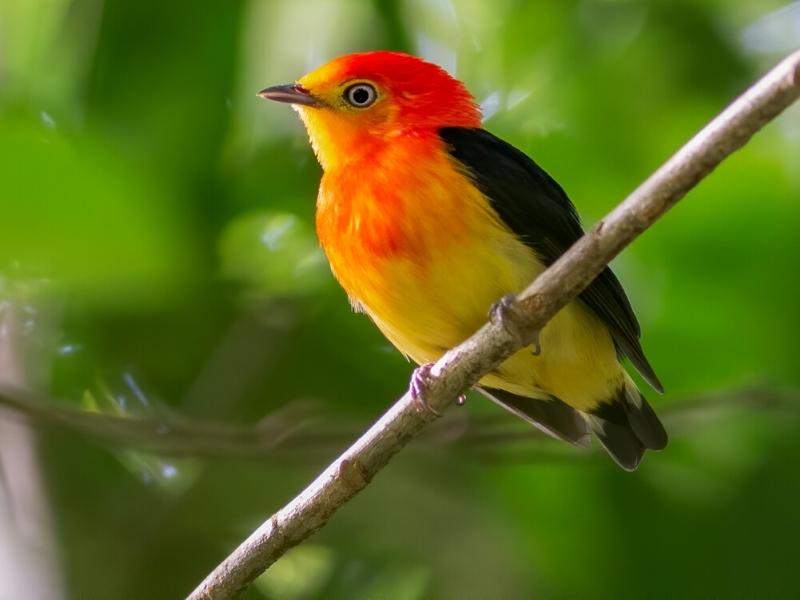In this highly detailed nature photograph, a vibrant bird is perched on a twig that diagonally spans from the bottom left to the upper right of the image. The twig, about the size of a pencil, is perfectly clasped by the bird's small claws. The bird, predominantly orange with a yellow breast, has an orange crown and is accented with blackish-brown wings and a tail. Its body and head are oriented to the left, with a short, pointed beak also directed leftward. The bird's left eye is clearly visible and appears to be looking directly at the camera, while the right eye is obscured. The entire composition is set against a blurry, green background suggestive of leafy foliage, enhancing the focus on the bird. This intricate detailing, combined with the bird's colorful plumage that includes patches of red and black, makes it a striking subject, potentially similar to a house finch. The photograph, evocative of professional wildlife photography like that seen in National Geographic, captures the serene and detailed beauty of this small bird in its natural habitat.